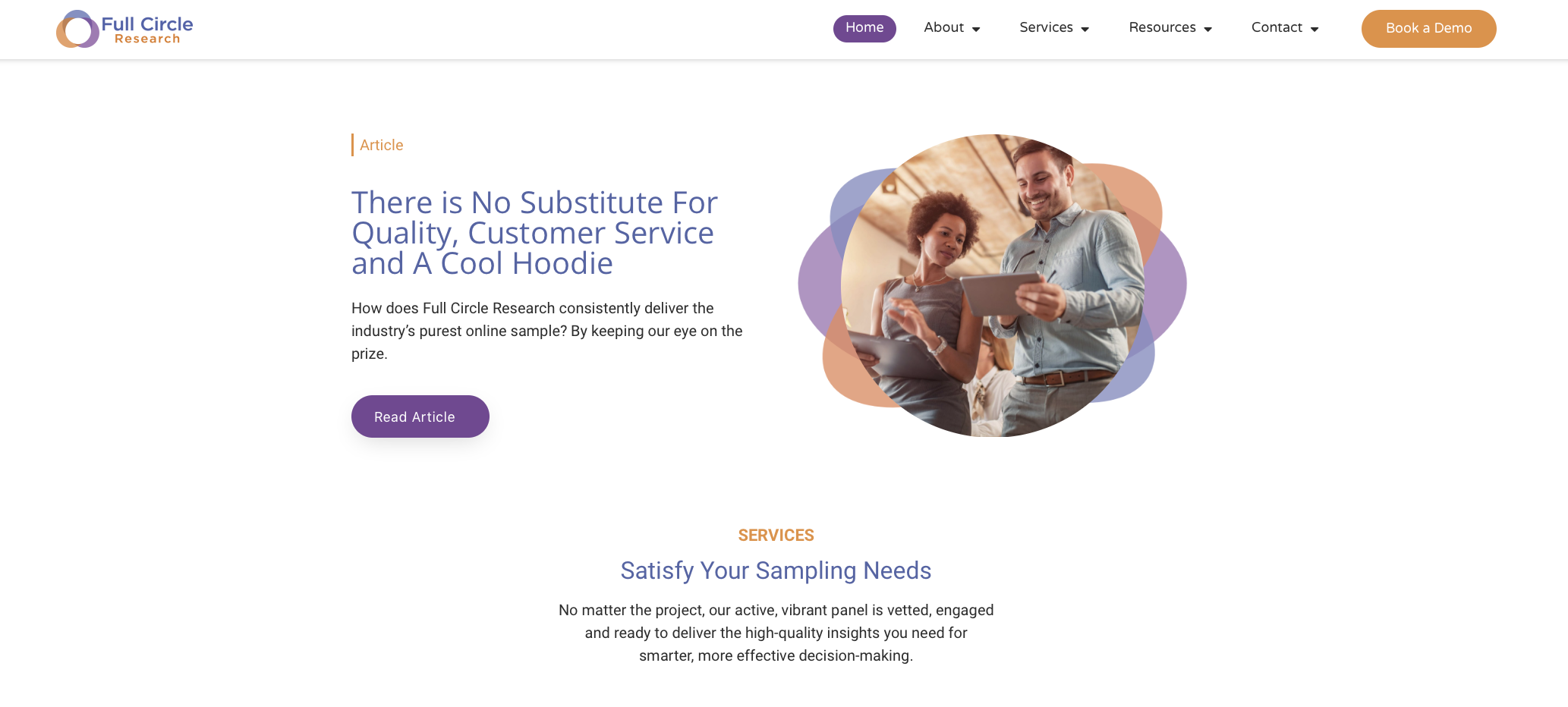This screenshot depicts a landscape-oriented webpage with a primarily white background. In the upper-left corner, the logo and name of "Full Circle Research" are displayed. The logo consists of a circular gradient transitioning from teal to purple to orange. The text accompanying the logo features "Full Circle" in blue and "Research" in orange. 

On the top right, there are several navigation tabs in a horizontal row, starting with a purple "Home" button, followed by "About," "Services," "Resources," and "Contact," each accompanied by a down arrow indicating dropdown menus. Additionally, an orange button labeled "Book a Demo" is positioned on the far right of the navigation bar, which sits atop a gray dividing stripe.

Below this header section, there is an image featuring two individuals, a woman and a man, standing in an indoor setting with a ceiling visible overhead. The woman has darker skin and curly hair, and she is wearing a gray t-shirt. The man, standing to her left, has slightly lighter skin, black hair, a black mustache, and a small goatee. He is dressed in a blue button-up shirt paired with a brown belt and pants. The woman between them in the background is wearing a white shirt. The woman on the left is focused on the man’s tablet, and she has her right hand raised, adorned with a bracelet. 

To the left of the image, a text box reads, "Article: There’s No Substitute for Quality Customer Service and a Cool Hoodie." Directly beneath this text, a purple button is labeled "Read Article."